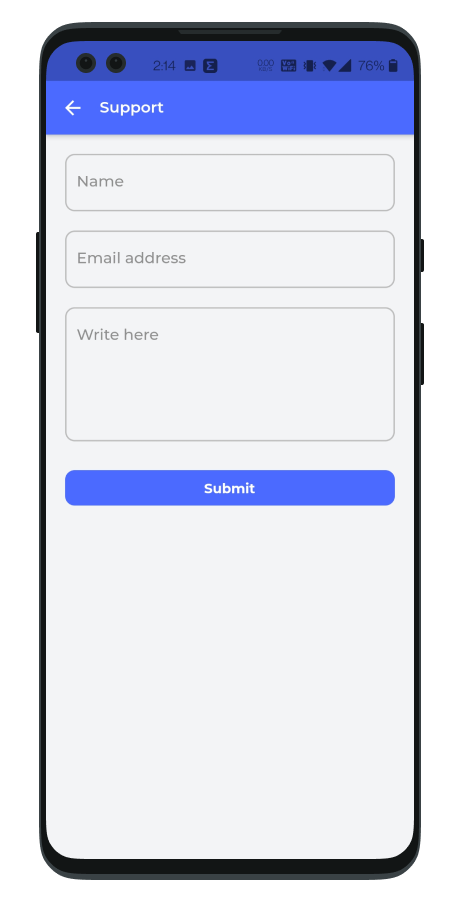The image showcases a detailed mock-up of a smartphone displaying an app interface. The smartphone has a black bezel encompassing the screen, featuring two buttons on the right-hand side and one large button on the left-hand side. At the top of the screen, several icons are present, along with dual black circle cameras centrally positioned. The time displayed is "214," suggesting military time format.

Below, there is a square indicating a screenshot, displaying a black background with white mountain icons. Adjacent to this is another square with a white "E" on a black background, followed by "ODO," or "0.00 KB/S," representing data transfer rates. Further to the right are indications for the type of data, marked as "VO."

The status bar includes a black phone icon with vibration lines signifying active vibration mode, a fully filled Wi-Fi signal, and a full cell phone signal. The battery icon, nearly full, shows a 76% charge. Below this, a light blue rectangle features a bold white left-pointing arrow and "SUPPORT" in bold white text.

The main interface is a login webpage with a light gray background. It displays three input fields: "Name" on the left inside the first rectangle, "Email Address" on the same side of the second rectangle, and "Comment Section" labeled "Right Here" in the larger third rectangle. Below these fields, a rectangular button with rounded corners is present, colored dark blue with "SUBMIT" in white text at its center.